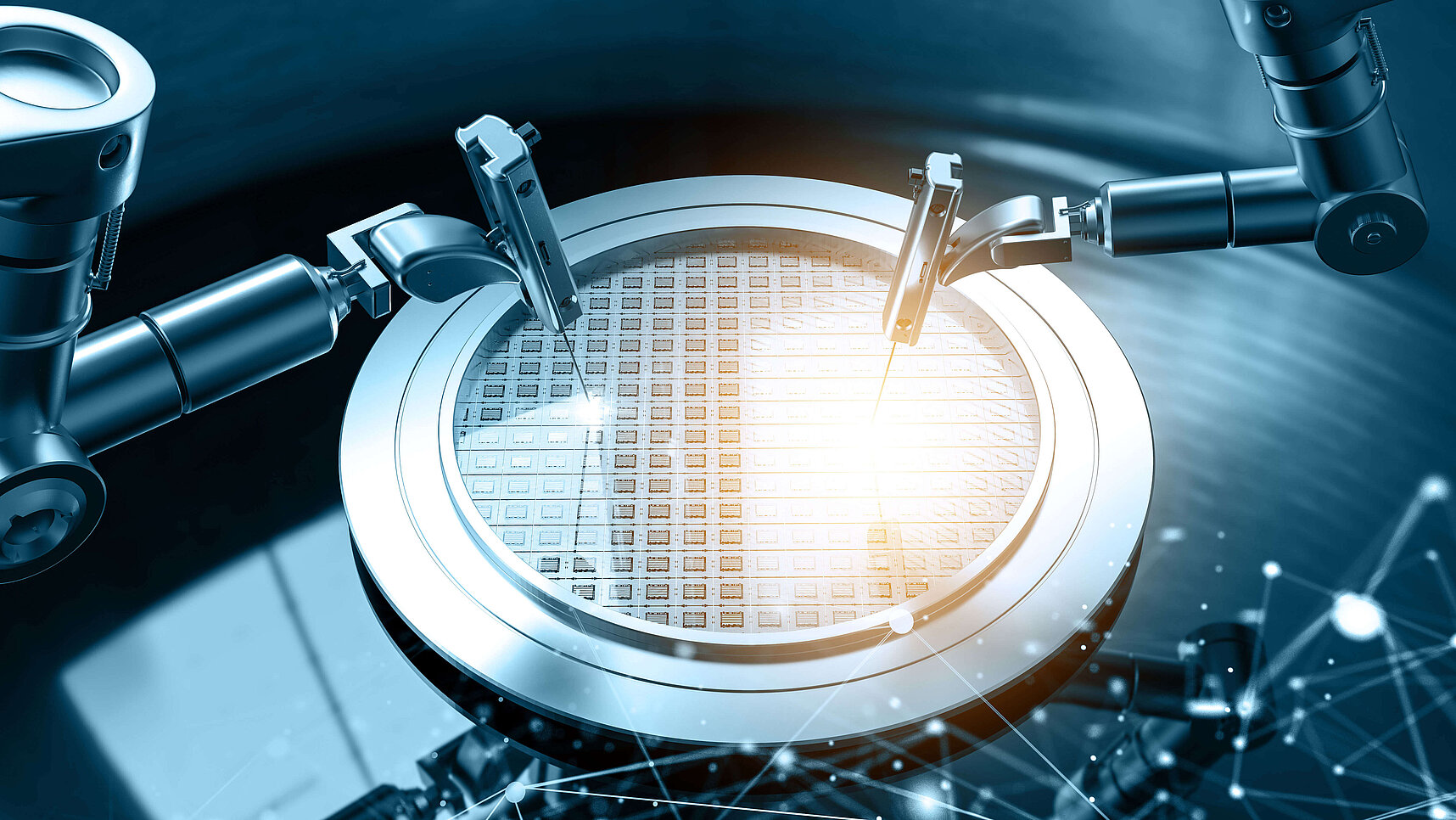This image, rendered in various shades of blue, showcases an intricate and futuristic scene featuring robotic arms engaged in a high-tech operation. These narrow, motorized arms descend from the top left and side, curving meticulously as they work with needlepoint precision on microchips or semiconductors, which are held within a circular retainer. The needlepoint tips of the robotic arms appear to be emitting bright lights, potentially for welding or lasering intricate patterns onto the microchips. The scene is lively with overlaid bursts, stars, and crisscrossing lights, creating a dynamic atmosphere of electronic component production. In the bottom left corner, there are bright, blurry white dots interconnected by thin lines, adding to the science-fiction aesthetic of the image. The overall palette ranges from very light blue to almost black, enhancing the futuristic and high-tech ambiance of this artist’s creation.